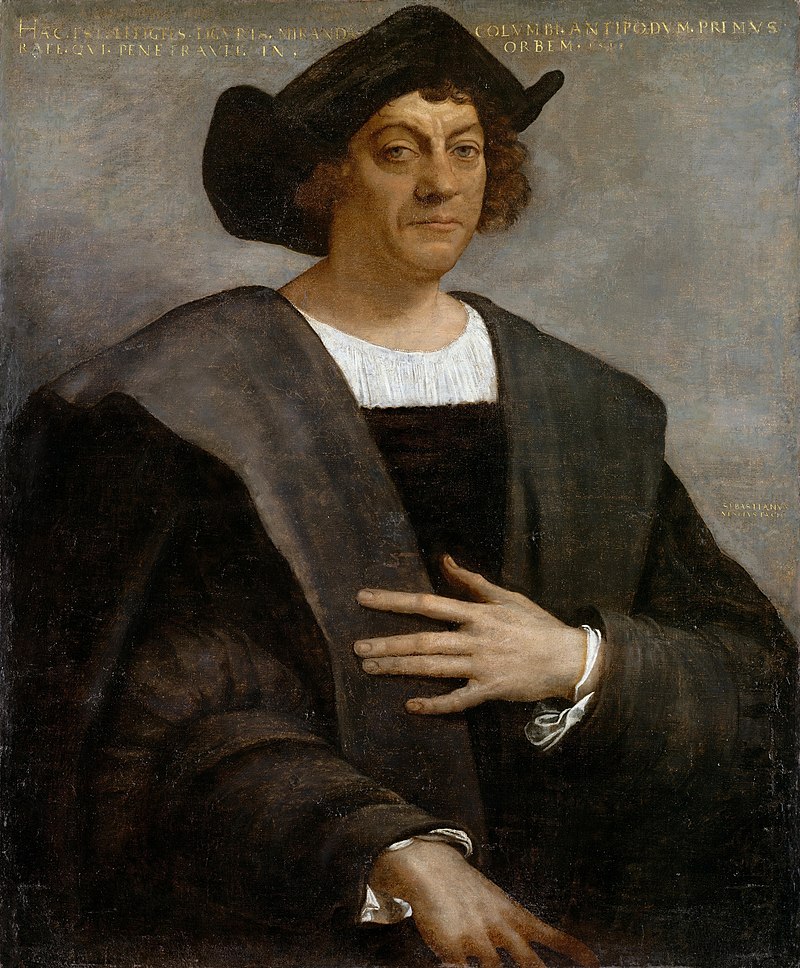The image depicts a meticulously detailed oil painting, appearing almost photograph-like, raising the question of whether it is a true oil painting or a digital illustration. The absence of a visible frame and the lack of discernible texture suggest it might be a modern digital rendition. The painting portrays a portrait from what seems to be an older historical period, possibly the era of Henry VIII.

The subject of the portrait is a man posed in a side-on stance, exuding an air of refinement and perhaps a hint of regality, though not necessarily of royal blood. He dons a unique triangular hat with a rounded tip, under which flows curly brown hair cascading down both sides of his face. His expression is solemn, marked by a curious detail—his left eye appears to wander towards the left corner while his right eye gazes straight ahead, suggesting a possible lazy eye or a quirk of the painting's style.

His attire consists of a white top with vertical ruffles around the neck, adding a touch of elegance. Draped over his shoulders is a substantial, heavy-looking shawl, which he clutches to his chest with his left hand. His right arm, adorned with wide, ruffled dark sleeves, rests on his leg, extending out of the frame at the bottom. The overall color palette of his clothing transitions into shadowy blacks, creating a striking contrast and emphasizing the depth and richness of his attire.